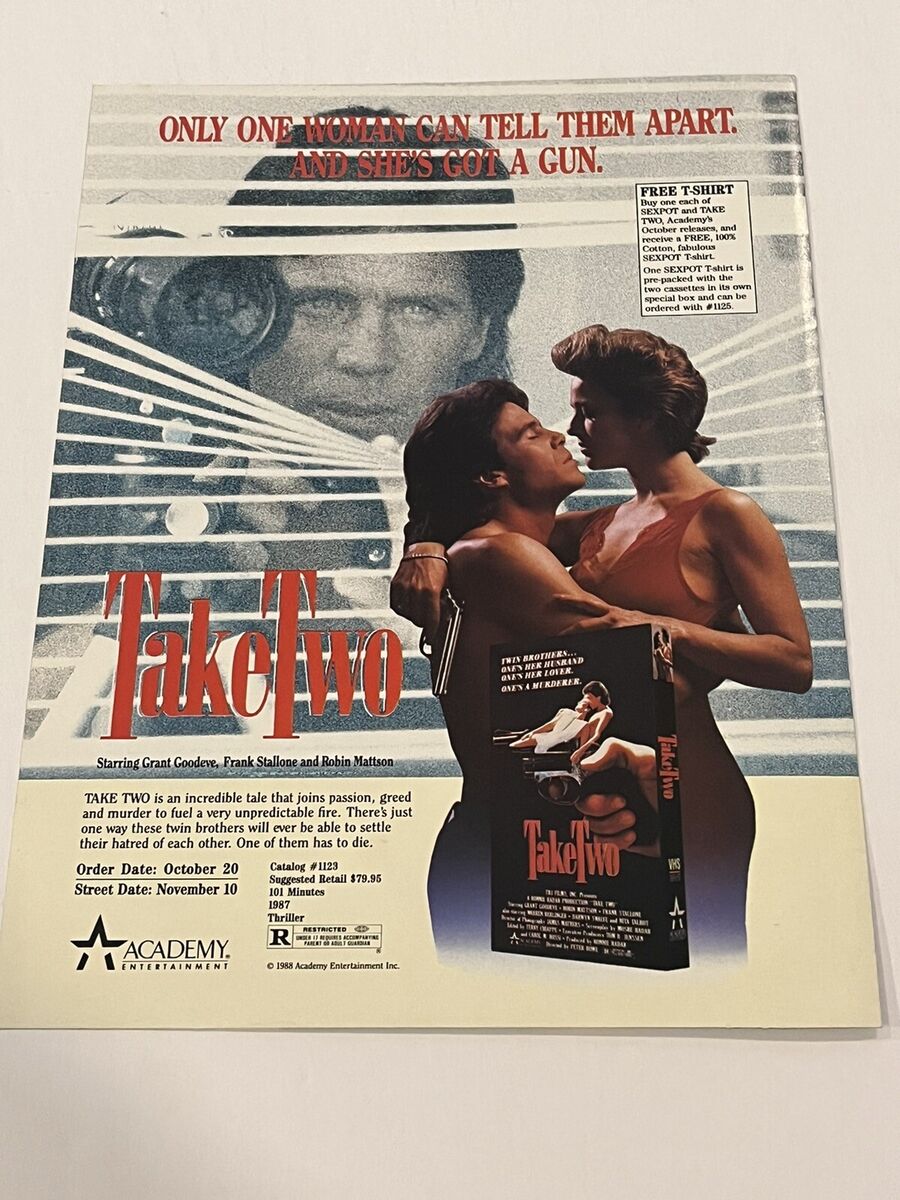This image showcases a portrait-oriented photograph of a full-page magazine advertisement for the movie "Take Two," likely released in the late 1980s. The ad, torn from a magazine and laid on a white table, prominently features a small isometric view of the VHS cover for the film. At the top of the page, in bold red capital letters, the tagline reads, "ONLY ONE WOMAN CAN TELL THEM APART AND SHE'S GOT A GUN." Below this, the central visual elements depict a dramatic scene: a shirtless man and a woman in red lingerie embrace, with her holding a gun in her right hand, pointing downward behind his back. 

In the background, a large grayscale image captures another man peering through Venetian blinds with a telephoto camera lens, suggesting an air of mystery and surveillance. Towards the bottom right of the ad, text provides additional information about the movie, including the order and street dates (October 20th and November 10th, respectively), inviting viewers to purchase their copy for home viewing. The tagline beneath the couple describes the movie as an "incredible tale that joins passion, greed, and murder to fuel a very unpredictable fire" with a climactic note about twin brothers where "one of them has to die." The movie stars Grant Goodeve, Frank Stallone, and Robin Mattson and is brought to you by Academy Entertainment.